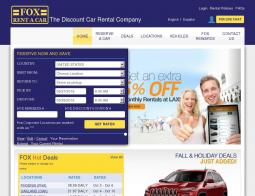The image depicts the homepage of Fox, an online car rental company. The brand name "Fox" is prominently displayed in yellow text on a blue background, inside a standalone box. The top section of the page features a navigation bar with several clickable categories, with the first category highlighted. Beneath the navigation bar, there's an information input form where users can enter their details to get started. Adjacent to this form is a yellow "Next" button. 

On the side of the form, there is an orange text message indicating a special offer, which appears to be a discount with a "5" at the end, potentially becoming visible once the information is entered and the "Next" button is clicked.

A large image showcases a cheerful man and woman taking a selfie. Below this image, there is detailed information about various car rental options. On the bottom right, an image of a red SUV crossover is prominently featured, suggesting this model is a highlighted promotion.